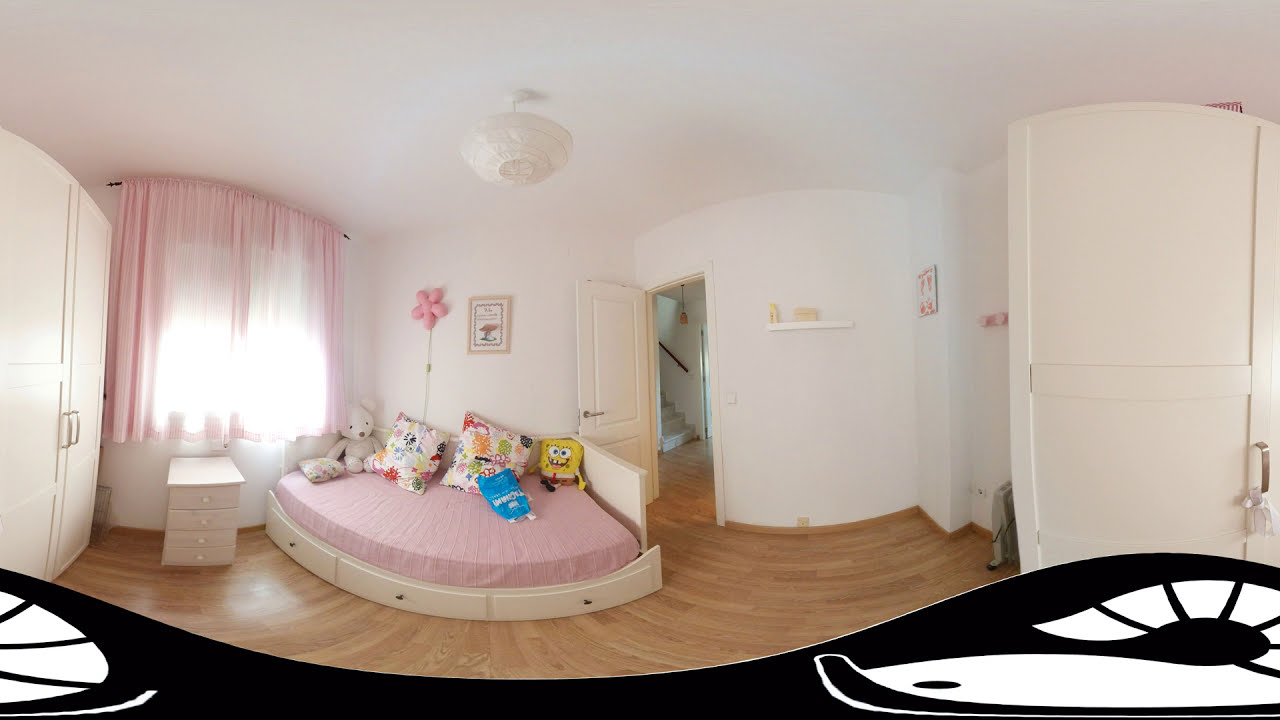The image depicts a meticulously clean child's bedroom with a bright and welcoming atmosphere. The room features light brown wooden flooring and predominantly white walls and ceiling, which enhance the natural lighting that filters through sheer pink curtains over a large window. Centrally, there's a white bed with a pink comforter positioned against the corner. The bed base features three beige dresser drawers, and it's adorned with two throw pillows and two stuffed animals, notably including a prominent SpongeBob SquarePants plush. To the left of the bed stands a large, plain white two-door armoire, while beneath the window is a small four-drawer white nightstand. On the wall behind the bed, a pink flower decoration and a photograph or painting add a touch of personalization. An open door at the foot of the bed leads to a brightly lit hallway with stairs ascending to the left. A ceramic white ceiling light fixture is centered at the top of the room, completing the tidy and harmonious setting.